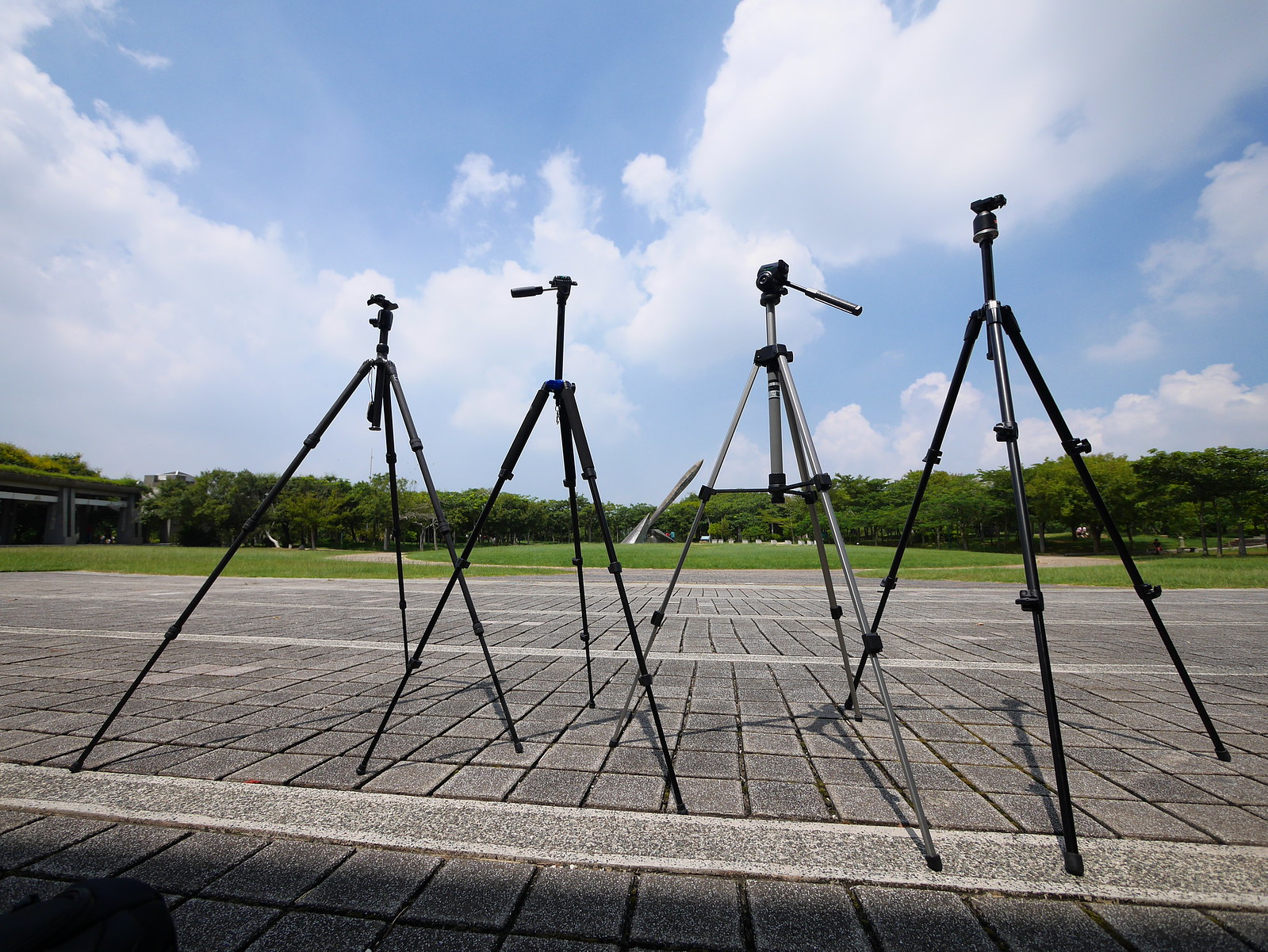This photograph captures a serene outdoor setting featuring four tripods set up on a paved patio. The patio itself is made up of small gray square tiles bordered by long rectangular stones. In the background, a scenic park-like area can be seen, showcasing a short grassy lawn encircled by lush, green deciduous trees. A building is visible on the left side of the image, adding an architectural element to the natural scene. High above, a beautiful blue sky dotted with large white clouds stretches across the upper part of the photograph. The tripods, which stand tall with their legs fully extended, are arranged side by side in the foreground. While three of the tripods are black, the third one from the left stands out with its gray or silver legs and vertical body. None of the tripods are equipped with cameras or other gear at the moment.